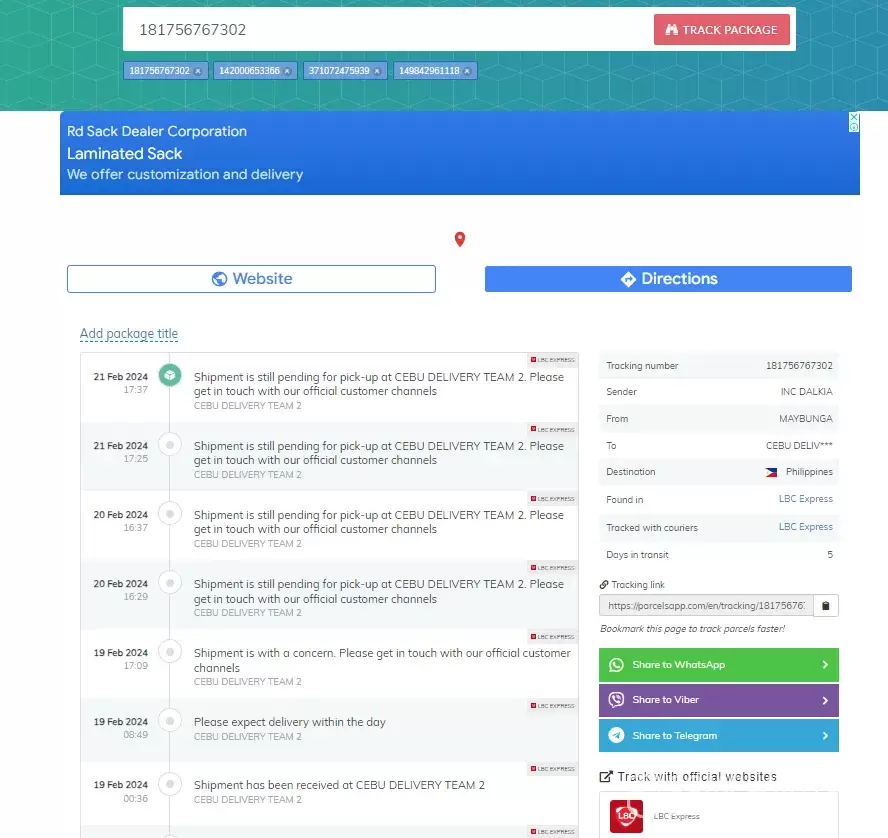This image depicts a webpage from a shipping website. At the top of the page, there's a prominent green bar and a search option. Below the green bar, a white input box allows users to enter their tracking number and press the "Track Package" button. This feature also saves previously entered tracking numbers for ease of future use. 

Below the tracking feature, the page is branded with "Road Sack Dealer Corporation - Laminated Sack." It also mentions that the company offers customization and delivery services. 

The webpage offers further functionalities such as seeking directions, adding a package title, and viewing tracking updates. The tracking information is displayed in a chronological list, with the most recent updates at the top:

1. **February 19, 2024**: "Shipment has been received at Cebu Delivery Team."
2. **February 19, 2024**: "Please expect delivery within the day."
3. **February 19, 2024**: "Shipment is with a concern. Please get in touch with our official customer channels."
4. **February 20, 2024**: "Shipment is pending for pickup at Cebu Delivery Team. Please get in touch with our official customer channels."
5. **February 2024**: "Shipment is pending for pickup at Cebu Delivery. Please get in touch with our official customer channels."
6. **February 21, 2024**: Two entries stating, "Shipment is pending for pickup at Cebu Delivery Team. Please get in touch with our official customer channels."

To the right side of the screen, additional details are provided, including the tracking number, sender information, origin, destination, courier service (LBC Express), and days in transit (which is five days in this instance).